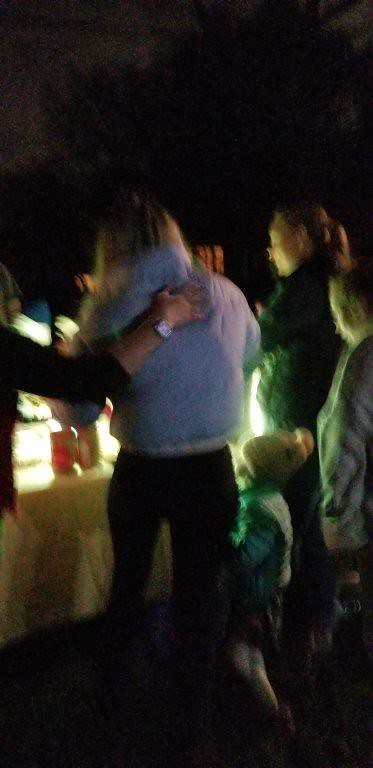In the blurry photograph, an outdoor nighttime winter social gathering unfolds in a dimly lit space. People are bundled in warm winter attire. Central to the image, a little girl clings to her mother's leg. The child wears a knit cap and a cozy jacket, while her presumed mother faces away from the camera, revealing long blonde hair and a winter jacket paired with black pants. An arm draped over the mother's shoulders, dressed in a dark sleeve rolled up to the elbow and sporting a silvery watch, suggests a masculine presence offering comfort or connection.

The group faces a well-lit table, illuminated by unknown light sources, possibly candles or lanterns. The table, draped in a white tablecloth, holds several unidentifiable items. To the right, another individual, likely female and dressed in a winter coat, gazes down at the table. Nearby, a third person with hair tied in a ponytail and clad in a green winter jacket completes the scene, contributing to the cozy yet mysterious ambiance of the gathering.